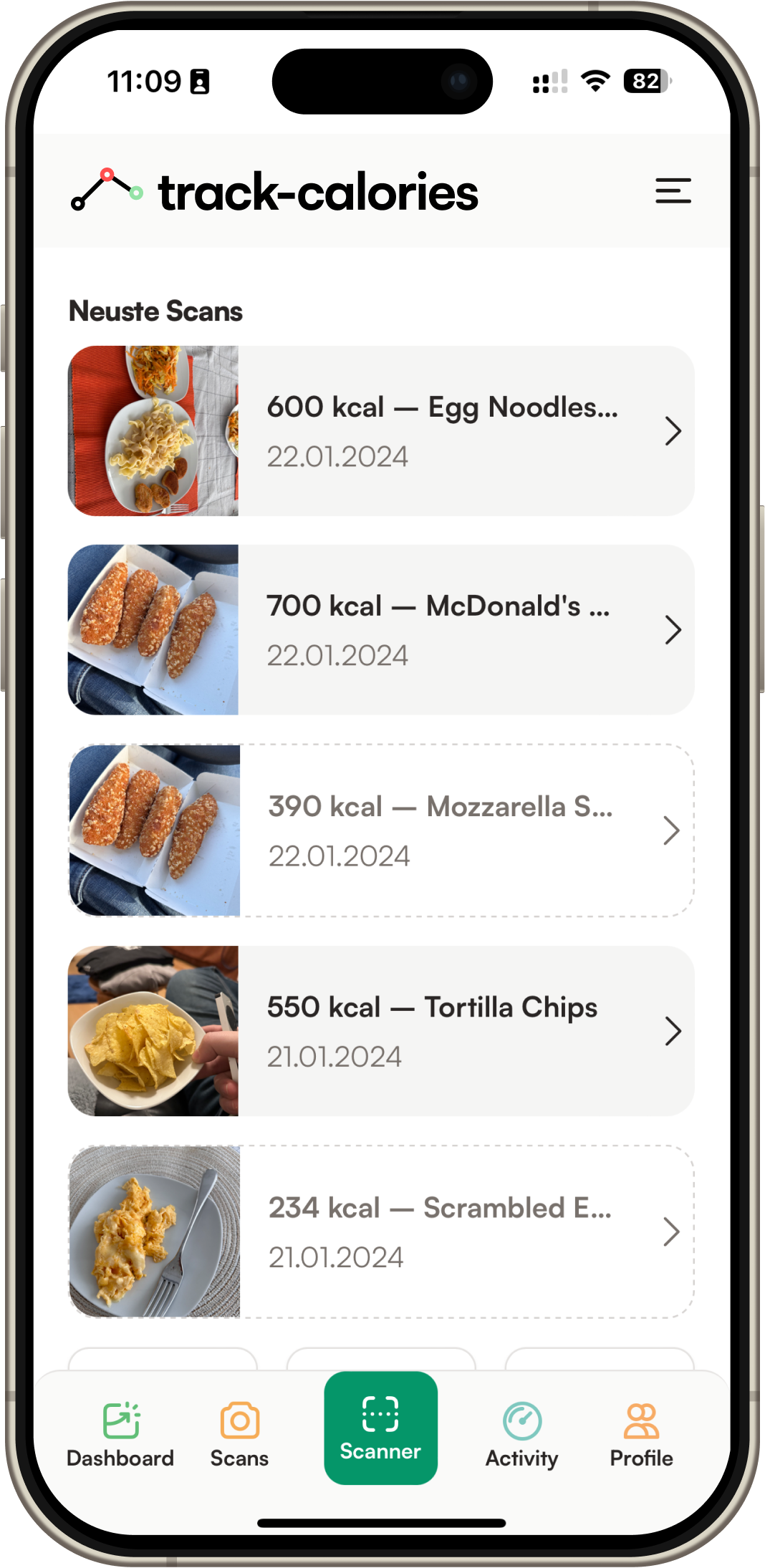This image showcases a screenshot of a calorie tracking app displayed on a smartphone. The app interface features a white background with the title "Tracked Calories" prominently shown in black font at the top. In the main content area, there are entries for five different meals, each accompanied by the dates they were consumed, the number of calories, and brief descriptions of the food items, such as egg noodles, McDonald's, tortilla strips, and scrambled eggs. On the left side of each meal entry, individual pictures of the respective food items are displayed.

At the bottom of the screen, there are five navigation options: "Dashboard," "Meals," "Scanner" (centered), "Activity," and "Profile." The device itself has a sleek design with curved edges and is connected to Wi-Fi, as indicated by the signal icons at the top right corner of the screen. The battery life of the smartphone is at 82%. The current time, displayed at the top left corner, is 11:09. The screenshot provides a comprehensive view of the app's functionality and the smartphone's interface.